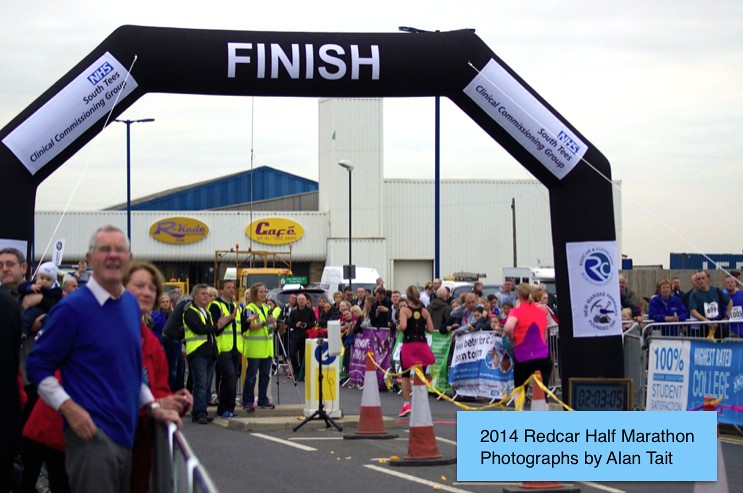The image captures a dynamic scene at the finish line of the 2014 Red Car Half Marathon, photographed by Alan Tate. The setting is an outdoor race course on what appears to be a hazy, yet cloudless, day. Dominating the center of the image is a black, trapezoidal inflatable structure with "FINISH" boldly written in white letters across its top. This serves as an archway through which runners are seen crossing.

In the foreground, two runners are completing the race. The first runner, attired in a black shirt and shorts, and the second in a vibrant purple and orange shirt, are captured from behind, emphasizing their final strides. To the left side of the image, a group of spectators stands behind a metal barricade, eagerly watching and cheering. Among them, some individuals appear to be previous participants still wearing their bib numbers. Notably, a couple in the foreground are distinguishable – the man in a blue shirt and the woman in a red shirt. Adjacent to the runners on both sides are orange and white traffic cones with ribbons delineating the race lanes.

A few race officials clad in lime green vests are seen clapping and encouraging the runners near the barricades. There's a notable signage below the finish line stating "100% student" and a partially readable phrase about a college. Behind the spectators, a white building with a yellow "Capco" sign is partially visible in the background. The bottom right corner of the image features text over a light blue background, clearly indicating “2014 Red Car Half Marathon. Photographs by Alan Tate.” The colors in the photo, including gray, blue, white, red, black, lime green, yellow, maroon, and orange, add to the lively atmosphere of this racing event.